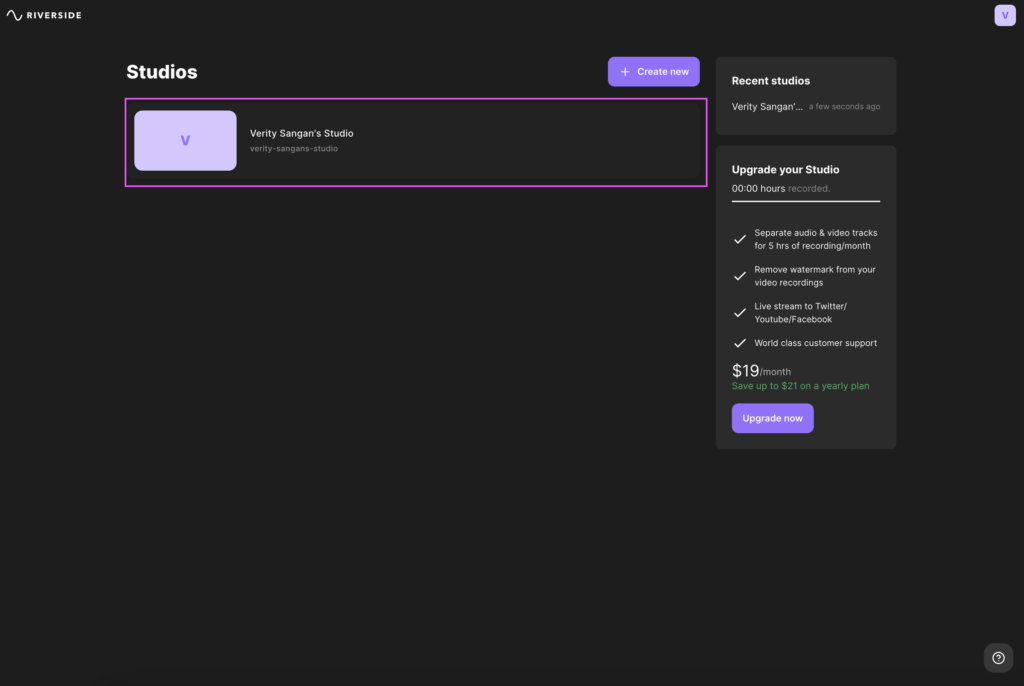The image is a screenshot from the Riverside website, recognizable by its distinctive sideways squiggly 'S' icon. "RIVERSIDE" is prominently displayed in bold, uppercase white letters on a solid black background. 

At the top of the image, there's a curved lavender box with a deeper purple letter "V" inside, complementing the monochromatic theme. Next to this box, in white print, are the words "Verity SsangYans Studio". Below this text, a secondary label reads "Verity-SsangYans-Studio". This section is outlined by a glowing purple rectangle, enhancing its prominence.

Underneath the outlined section, there's a clickable purple box labeled "+ Create New," signifying an option to create a new studio. To the right, under the heading "Recent Studios," is a recent entry: "Verity-SsangYan," followed by ellipses and a timestamp indicating it was updated "a few seconds ago."

Further down, there's another section titled "Upgrade Your Studio." This segment indicates there have been "00:00 hours recorded" so far. At the bottom, pricing details are highlighted: "$19 a month" with a green note emphasizing the potential savings—"Save up to $21 on a yearly plan." Adjacent to this, a purple "Upgrade Now" box invites users to purchase the plan.